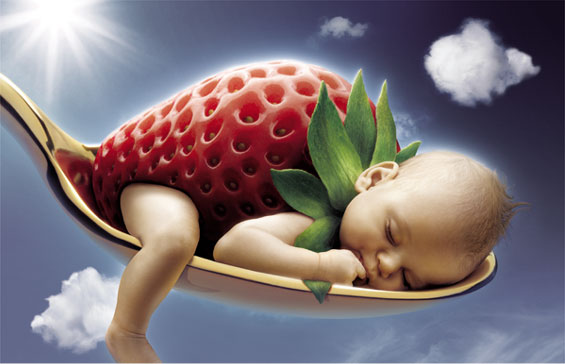In this whimsical fantasy image, a peculiar baby peacefully slumbers with a finger in its mouth, nestled comfortably in the bowl of a spoon suspended against a backdrop of a vibrant blue sky dotted with fluffy white clouds. The child has a delicate fuzz of fair hair and an unusual body resembling a large, ripe strawberry. The vivid details of the strawberry are striking, with its tiny pitted seeds clearly visible across its surface. From this berry-like body, the baby's arm and leg extend naturally. Around the child's neck, a green calyx rests like a quaint collar, adding to the surreal combination of human and fruit. This charming fusion gives the impression that the child is either snugly enveloped in a strawberry suit for warmth or is an enchanting blend of human and strawberry. The overall scene exudes tranquility and a sense of wonder.